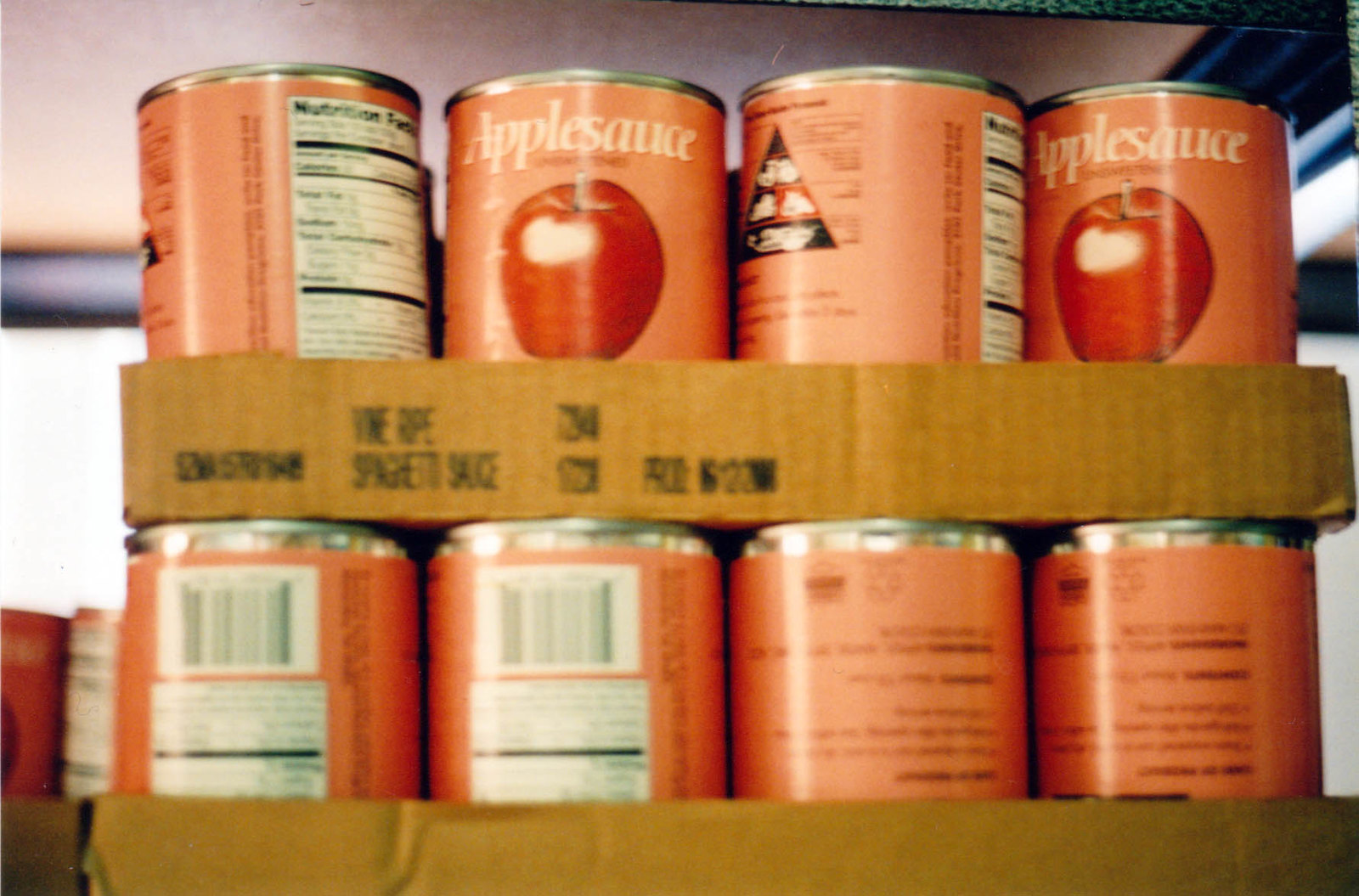A small cardboard box, approximately an inch tall and light brown in color, houses two stacked layers of canned fruit. Each layer contains four aluminum cans with pinkish labels, prominently featuring a red apple and the word "applesauce." The cans are in disarray; some face forward, while others are sideways or even upside down, displaying their UPC codes and nutritional information. Notably, one can near the middle-right side features a unique pyramid design interspersed with indistinguishable drawings and reflections of light. The background is blurred, revealing a white ceiling and walls that hint at additional storage or groceries.